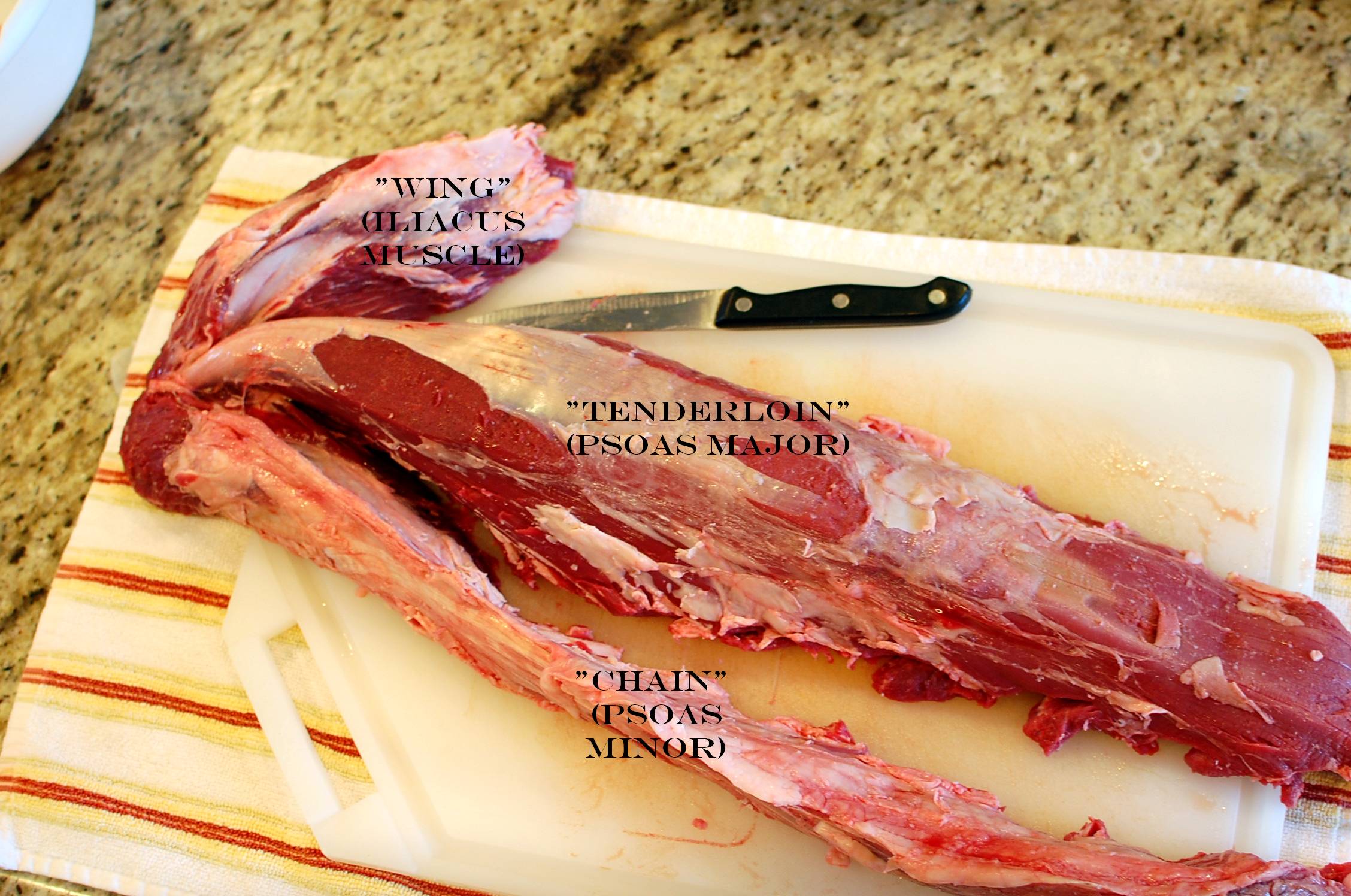The image depicts a raw piece of meat, potentially beef or deer, meticulously laid out on a white plastic cutting board stained with blood. The cutting board rests on a speckled yellow and brown countertop, accompanied by a white kitchen towel featuring yellow stripes with an orange stripe down the middle. To the left, the tip of a white bowl is partially visible. The cutting board itself, rectangular with a cut corner forming a handle, hosts a large, red-brown piece of raw meat that has been partially carved and spans across the entire surface, spilling over the edges.

Each section of the meat is labeled with both common and scientific names. The top portion is marked "wing" along with another label term not fully visible, suggesting it might be the "callous muscle." The central, main segment of the meat is labeled "tenderloin" (Psoas major), and the bottom part is marked "chain" (Psoas minor). A black-handled knife lies above the middle section, hinting at ongoing preparation. The raw meat's bright red color and clinging fascia-like material highlight its uncooked state, while the bone within gives hints of white, emphasizing the meat's fresh and unprocessed nature.